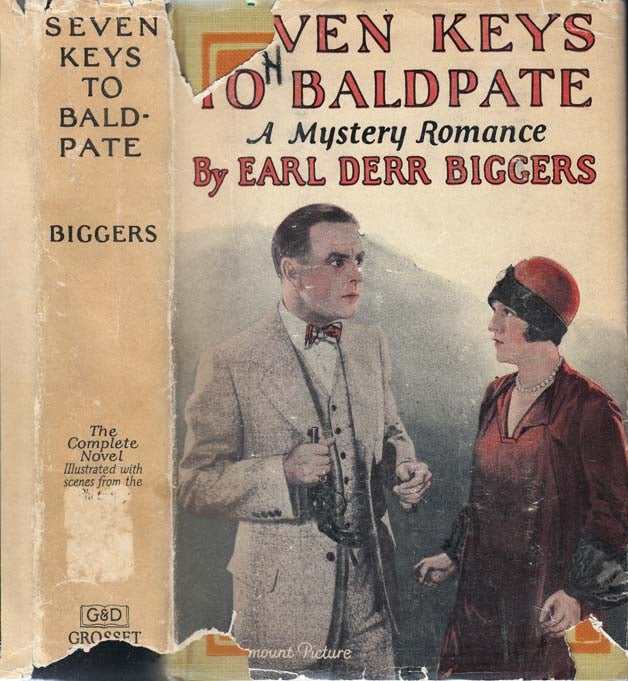The image features a worn and torn antique book cover of "Seven Keys to Baldpate: A Mystery Romance" by Earl Derr Biggers. The cover shows significant damage, with rips affecting the book's title; notably, the "S" and "E" of "Seven" are missing. The spine is partially ripped, and the paper has a weathered look. 

The top left of the cover reads "Seven Keys to Baldpate," followed by "Biggers." Below that, it states "The Complete Novel Illustrated with Scenes from the," but much of this text has been rubbed off. The bottom left corner mentions "Paramount Picture" and "G&D Grosset," though the latter part is also damaged. 

The central illustration features a scene from the 1920s, depicting a man and a woman in a moment of confrontation. The man, dressed in a light beige three-piece suit with a bow tie and wielding a pistol by the barrel, stands on the left. Opposite him is a woman in a red dress and a dark red beret, her dark black hair flowing from underneath. The interaction suggests tension, with the man appearing upset.